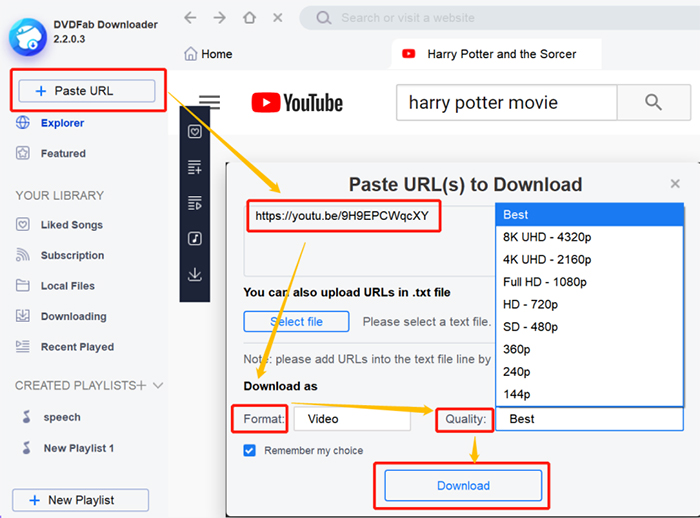Screenshot of the DVDFab Downloader Interface:
The image captures the DVDFab Downloader interface in detail. On the upper left-hand side, directly beneath the DVDFab Downloader icon, there is a prominently highlighted "Paste URL" button situated at the top of a vertical menu. Surrounding this button is a vivid red box, indicating its importance. A yellow arrow extends from this red box to a section labeled "Paste URLs to Download," which contains a specific URL for YouTube. Further guiding the workflow, another yellow arrow points from this section to a "Format" button. The "Format" button is similarly linked by a yellow arrow to a "Quality" button. Lastly, the "Quality" button is connected by a final yellow arrow to a "Download" button. These visual cues collectively define the sequence for downloading content using DVDFab Downloader.